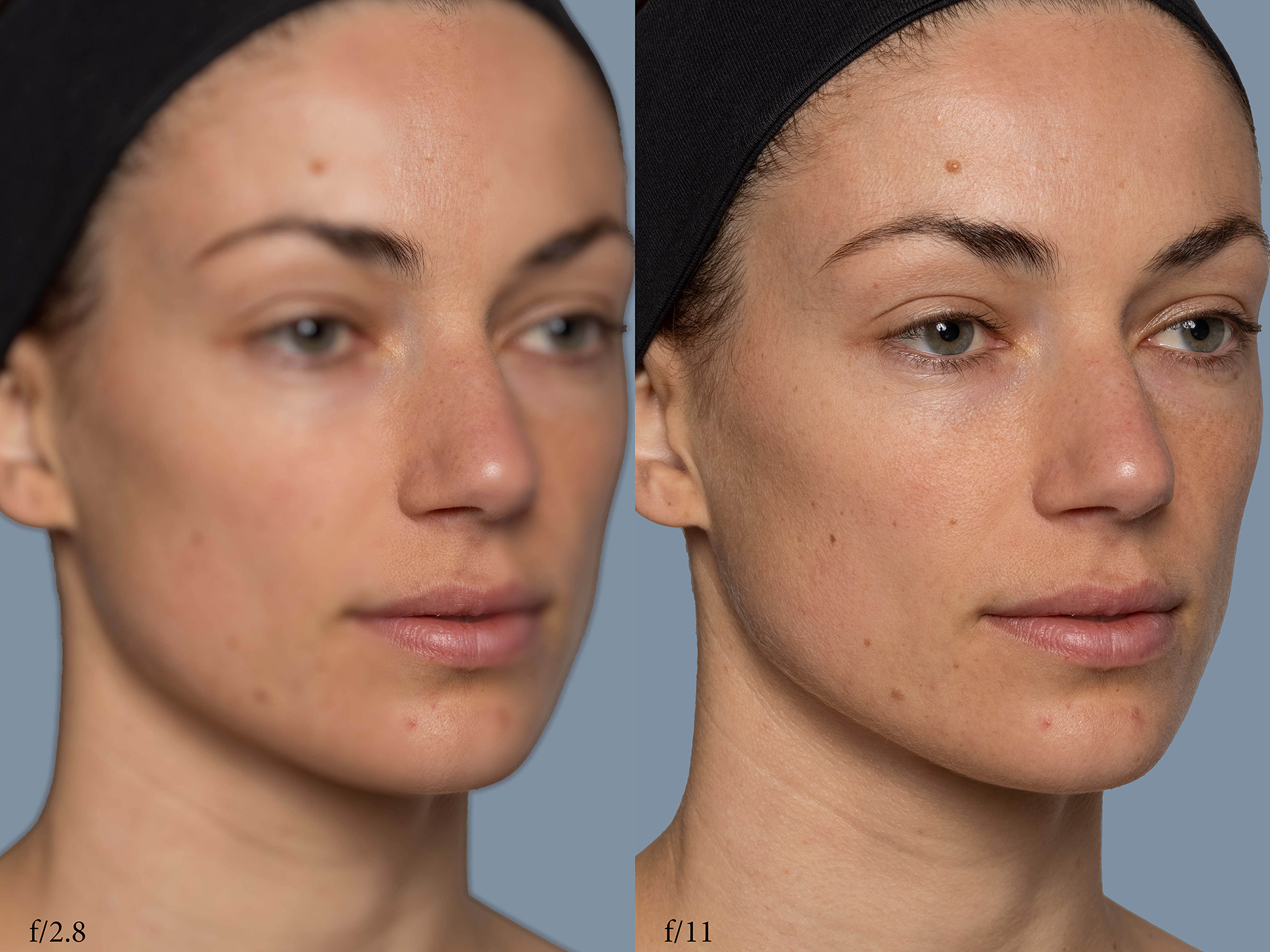The image is a large square picture showing a side-by-side comparison of the same woman's face, likely illustrating a difference in camera focus settings. On the left side, the image is blurry and marked "f/2.8" in the lower left corner, while the right side is in sharp focus and marked "f/11" in the corresponding corner. Both photos feature the woman looking slightly to the right with her lips slightly parted. She has a couple of freckles and a mole above her right eyebrow. Her eyes are depicted as either gray or green, and she is not smiling. The woman has a tight-fitting black cap or headband on, with some brown or black hair peeking out. The background of both photos is a grayish blue. There are small moles or discolorations visible around her chin and above her eye, and she has a slight blemish on her forehead. The main difference between the two images lies in the focus, with the details of her complexion, eyes, and facial features much clearer and more defined on the right-side image.